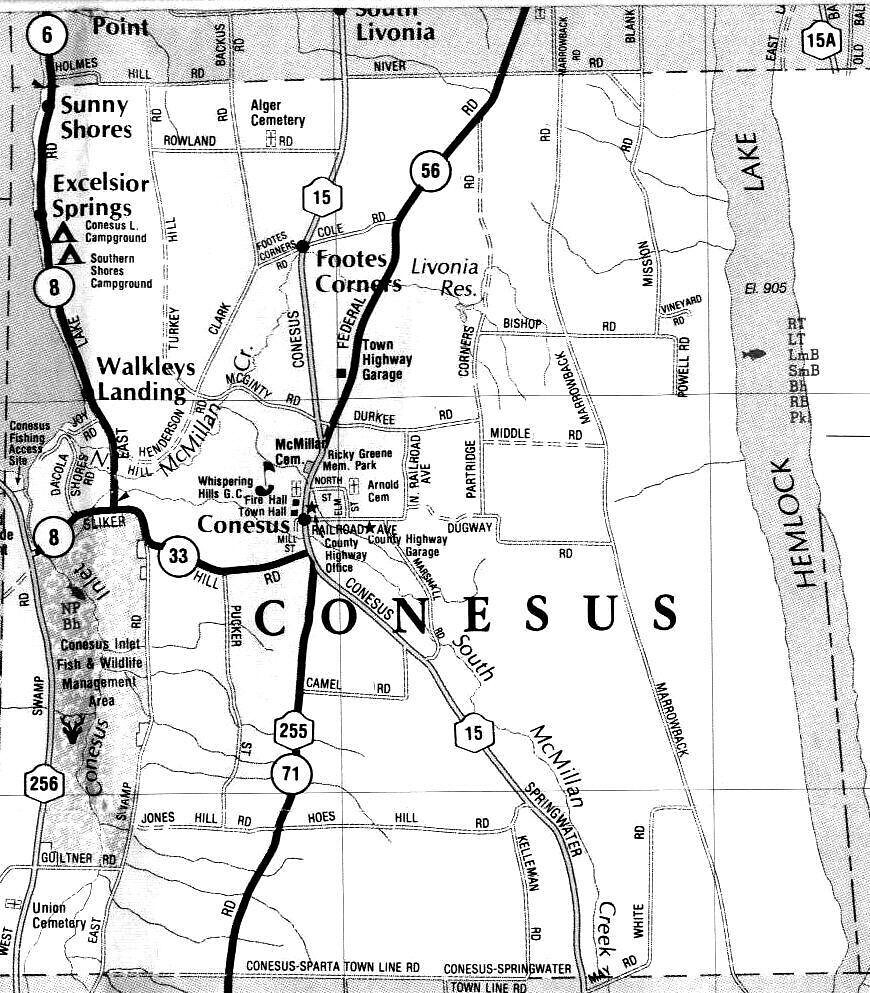A black and white map prominently features the city name Conesus (C-O-N-E-S-U-S) slightly off-center. To the right, a vertical waterway titled Hemlock Lake is adorned with a fish icon, stretching across the map vertically. The area is crisscrossed by various major routes and interstates including 56, 6, 8, 33, 71, 15, 255, and 256, with Route 56 primarily running north-south. A notable town center is marked by a black dot about halfway up the map. In the bottom left corner, Union Cemetery is labeled, while the top left corner highlights Sunny Shores and Excelsior Springs. The map exhibits a denser road network towards the central city area, with Route 56 transitioning into 15 around the center and Route 255 transforming into 33 at its intersection with Route 56 and 15. South Livonia and Foots Corners are also noted among the various local landmarks.